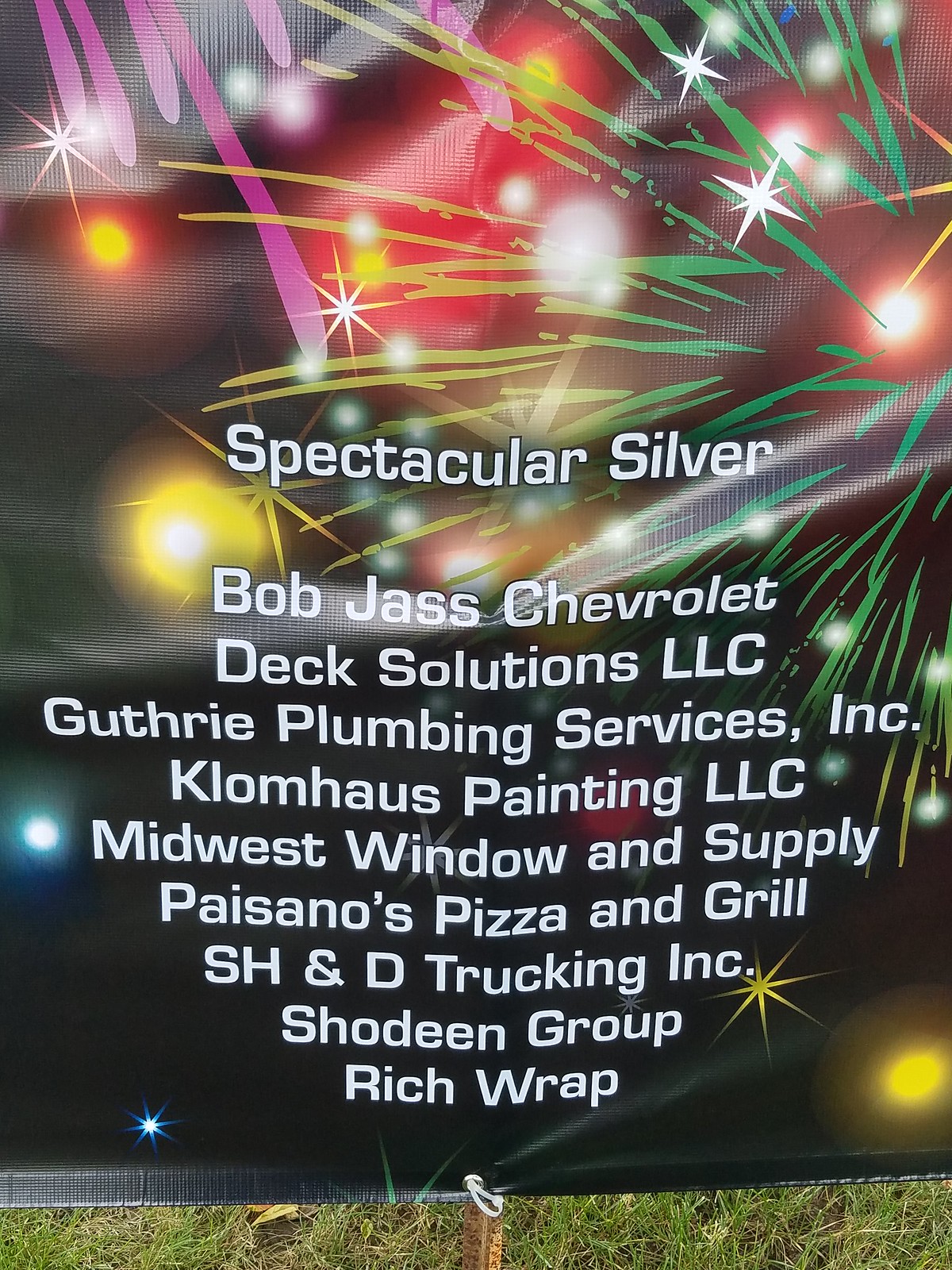This vibrant vertical rectangular poster looks like an advertisement for an event, featuring a dark black background that contrasts with a colorful explosion of fireworks and star-like patterns in shades of blue, yellow, green, red, fuchsia, purple, and orange. The lively colors and patterns resemble a mix of Christmas lights and grass, adding an energetic and festive feel to the image.

The top of the poster highlights the event’s name, "Spectacular Silver," in eye-catching white text. Beneath this headline is a list of sponsoring companies, including:

- Bob Jass Chevrolet
- DEC Solutions, LLC
- Guthrie Plumbing Services Incorporated
- Klum House Painting, LLC
- Midwest Window and Supply
- Paisano's Pizza & Grill
- SH&D Trucking Incorporated
- Schroding Group
- Rich Wrap

The bottom of the poster appears to be secured to a wooden stand embedded in grass, emphasizing the outdoor setting. This visually rich banner, tied to its support, seems perfect for drawing attention at a lively event or celebration.